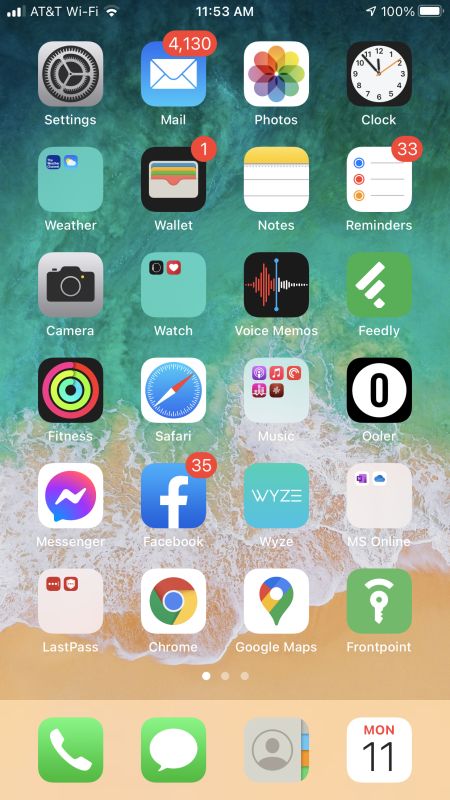A detailed image caption for a smartphone screenshot:

The image captures a smartphone screen displaying a clear and organized app layout. At the top of the screen, essential status indicators show 3 bars of network signal out of 4, connected to AT&T Wi-Fi, the time at 11:53 AM, and a fully charged 100% battery. Below these indicators, the main screen is filled with six rows of icons, each consisting of four apps. 

The apps from the top left to bottom right are:
1. Settings
2. Mail - displaying a red notification badge with 4,130 unread messages
3. Photos
4. Clock
5. Weather
6. Wallet - showing one unread notification
7. Notes
8. Reminders - highlighting 33 pending reminders
9. Camera
10. Watch
11. Voice Memos
12. Feedly
13. Fitness
14. Safari
15. Music
16. Ullr
17. Messenger
18. Facebook - with a notification badge showing 35 unread messages
19. Wise
20. MSOnline
21. LastPass
22. Chrome
23. Google Maps
24. Frontpoint

The screen is meticulously organized, providing a glimpse into the user's range of frequently used applications and pending notifications.